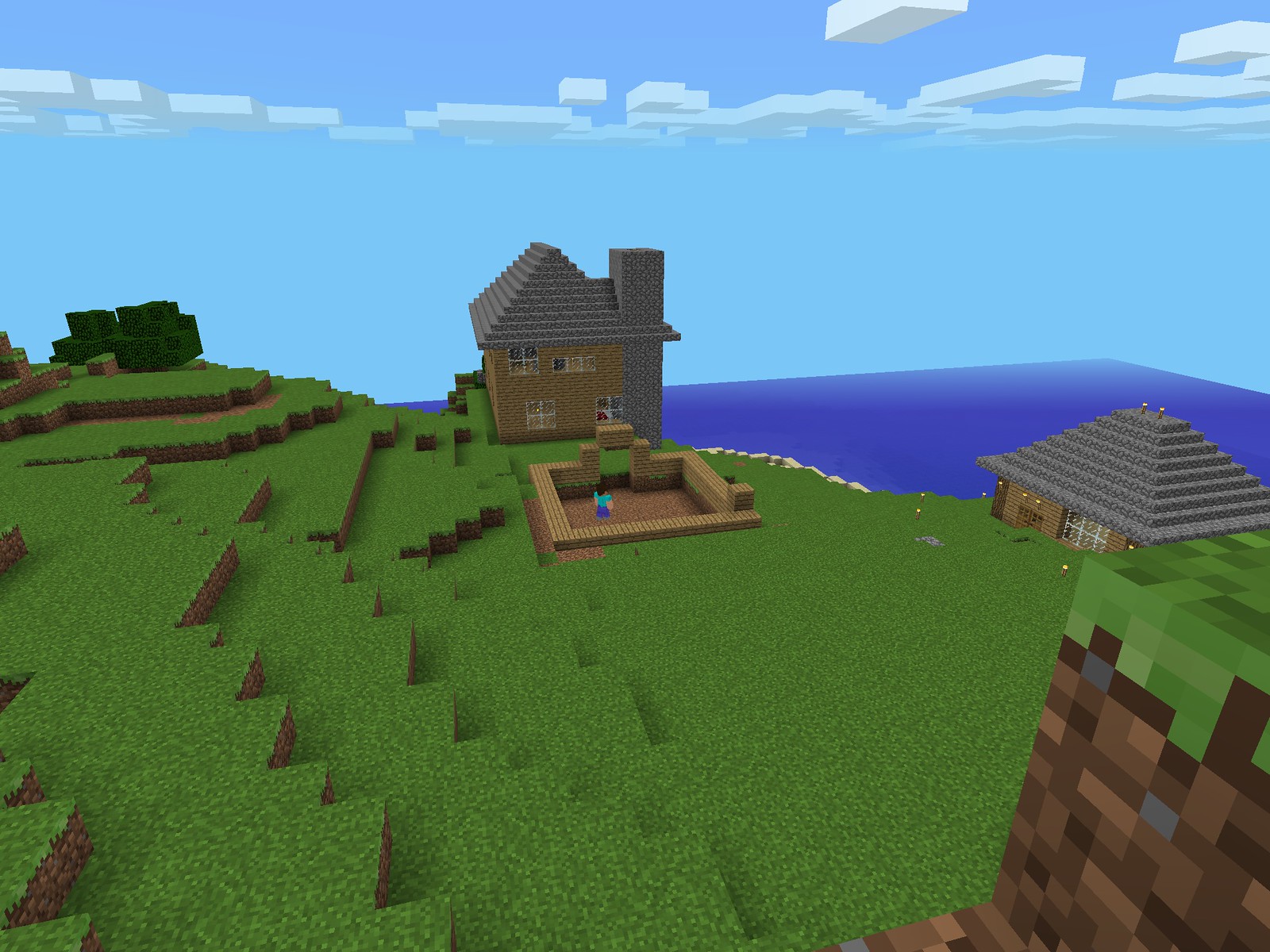The image resembles a scene from Minecraft, featuring a pixelated landscape that transitions from large, coarse pixels at the lower right to finer, detailed pixels towards the center. At the center of the scene, lush greenery represents grass. A character is visible alongside the foundation of a building, where the topmost layer appears constructed from brick-like materials. The central structure is a two-story building with a gray roof that slopes towards the middle. Adjacent to this, another building with a visible window suggests a single-story structure, its roof converging to the center from four sides. The setting seems to be on a hillside, with water visible in the upper right corner. The sky transitions from light teal to light blue, dotted with white clouds and tinges of black, while the upper left area shows more greenery, indicative of plant life or similar features.